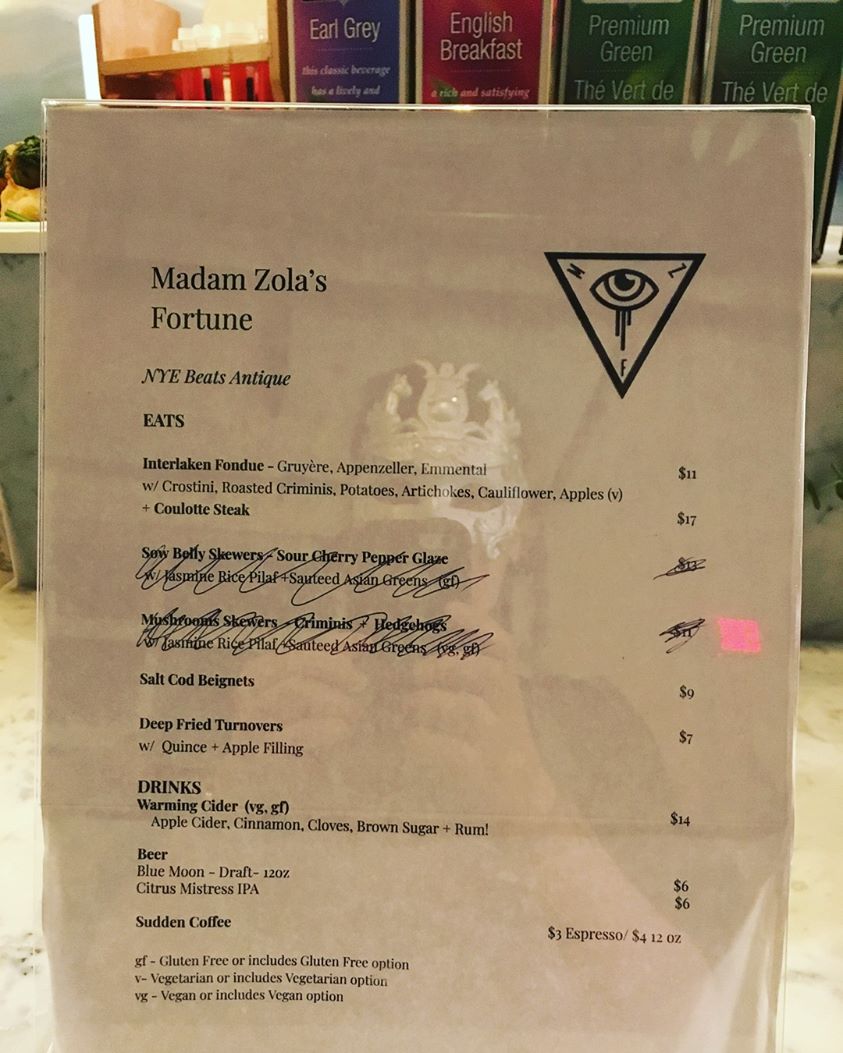This photograph depicts a simple, typed menu, encased not in lamination but likely protected by a plastic document wallet, commonly referred to as a "slippery fish." The menu itself appears to serve a dual-purpose venue, known as "Madame Zola's Fortune," where patrons can indulge in fortune-telling services while enjoying a meal. 

In the top right corner, the menu features a distinctive logo—a downward-pointing triangle containing an "I" shape with the letters "N," "Z," and "F" in each corner, representing the name of the establishment. 

The menu offers a variety of intriguing options:
- **Intertaken Fondue**: A rich blend of Gruyere, Appenzeller, and Emmental cheese, served with crostini, roasted cremini mushrooms, potatoes, artichokes, cauliflower, and apples. Priced at $11, or $17 with the addition of a culotte steak.
- **Unavailable Items**: A couple of selections have been crossed out, indicating their unavailability for the day.

Additional highlighted dishes include:
- **Salt Cod Beignets**: Priced at $9.
- **Deep-Fried Turnovers**: Filled with quince and apple, priced at $7.

The drink offerings are equally compelling:
- **Warming Cider**: A concoction of apple cider enhanced with cinnamon, cloves, brown sugar, and rum, priced at $14.
- **Draft Beer Options**: "Blue Moon," a 12-ounce draft beer for $6 and "Citrus Mistress," an IPA also priced at $6.

For coffee aficionados, "Sudden Coffee" comes in at $3 for an espresso and $4 for a 12-ounce cup.

The menu also includes a key for dietary preferences and restrictions, indicating gluten-free, vegetarian, and other dietary options. This straightforward yet charming menu offers a glimpse into the unique experience at Madame Zola's Fortune, blending culinary delights with the mystique of fortune-telling.